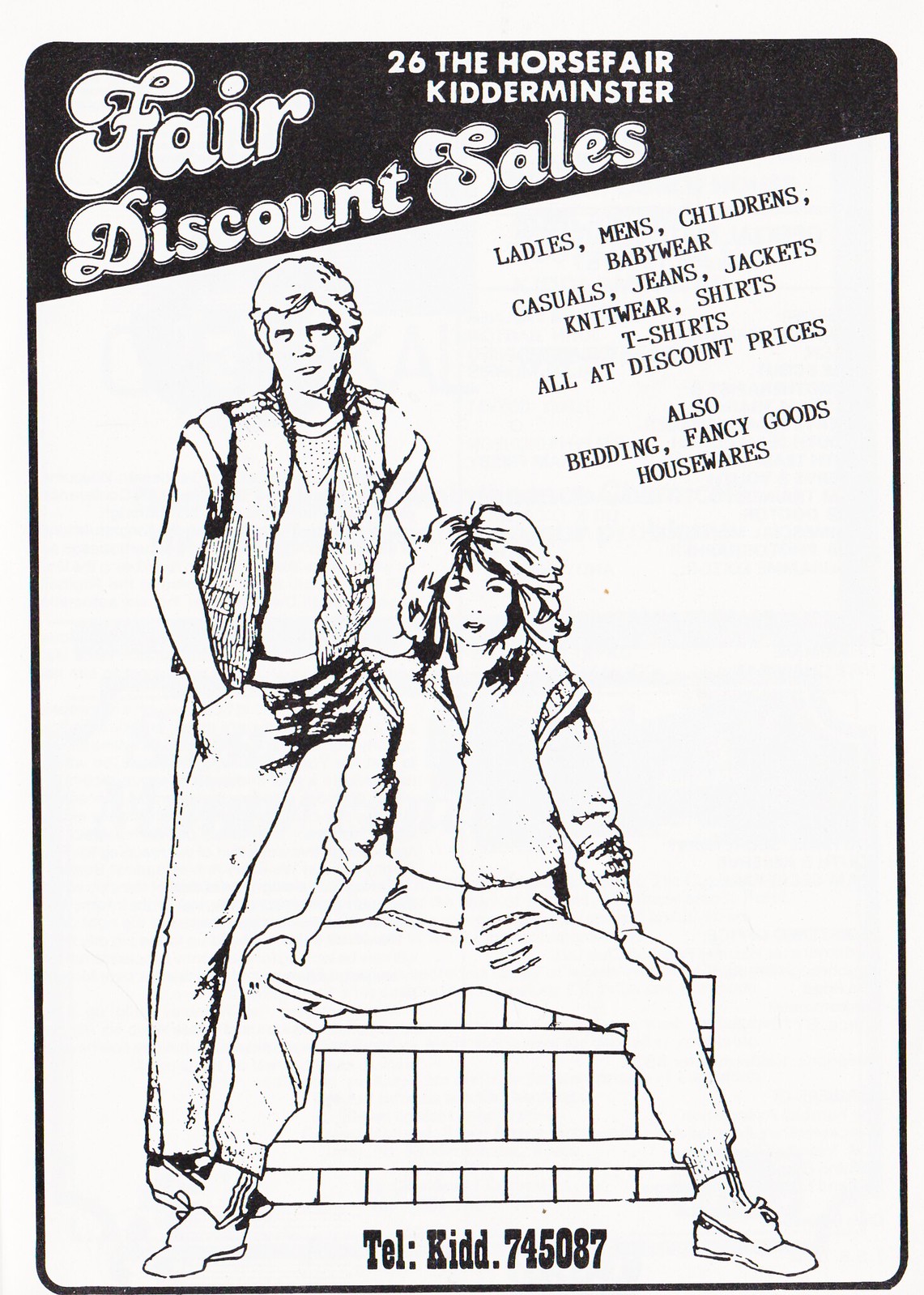The scan reveals a vintage black-and-white advertisement with a distinct black banner at the top. Displayed prominently in regular text, it announces the "26th Horse Fair, Kitterminster". Below, it declares "Fair Discount Sales”. The advertisement features an illustration of a stylish young man and woman, indicative of fashions from the late 70s or early 80s. The man, dressed in a vest with rolled-up short sleeves and hands in his pockets, stands behind the woman. She, with her flared hair and a jacket featuring flared shoulders, is seated on a wooden box, with her legs apart. To the right, an extensive list advertises "Ladies, Men, Children, Babywear, Casual Jeans, Jackets, Knitwear, Shirts, T-Shirts. All at discount prices" along with products like "bedding, fancy goods, and housewares". At the bottom, a contact number "tel: Kid 745087" is presented. The advertisement encapsulates what appears to be a department store sale, reminiscent of retailers like Sears or J.C. Penney, framed by a black outline with contrasting black and white sections across the image.